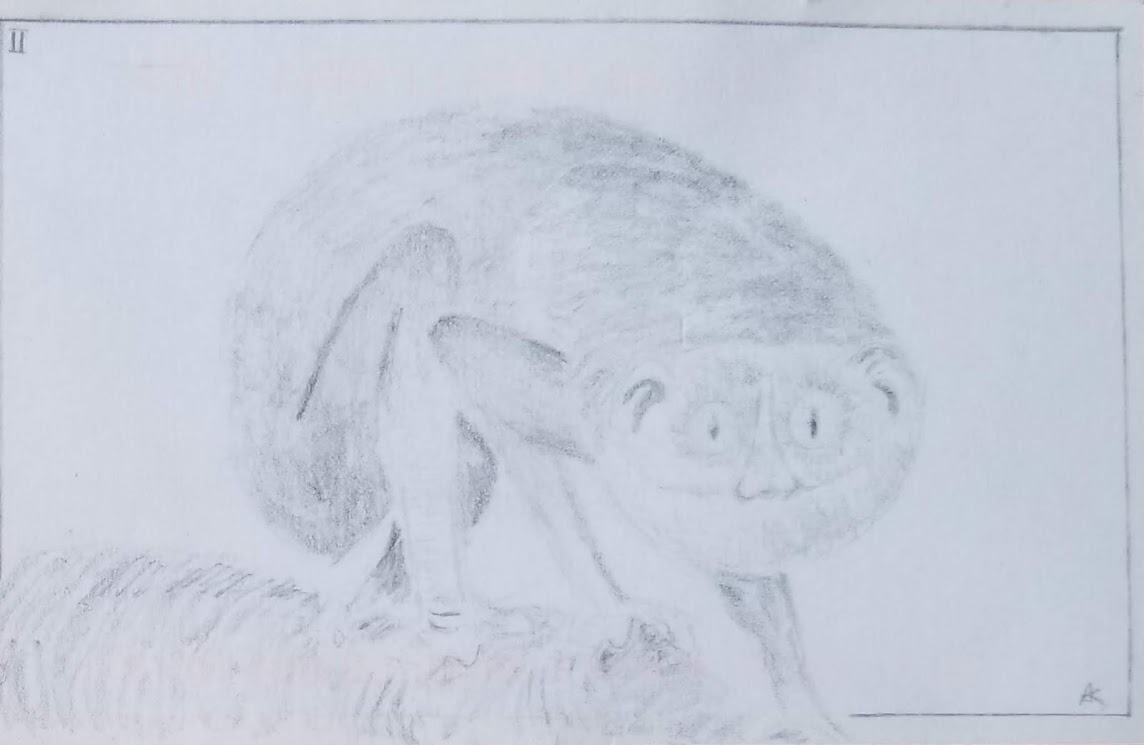This pencil drawing, set against a gray background, depicts an ambiguous four-legged animal resembling a sloth but not accurately rendered. The sparse, delicate strokes contribute to its ethereal and unclear presentation. The animal possesses disproportionately sized, wide eyes, with the left eye being larger. Dark areas sporadically accentuate parts of the animal, emphasizing the sketch's rough nature. 

The creature's body is rounded, with thin, slightly bent legs. Two back legs are visible, while one front leg rests on a small hill-like structure and the other remains grounded. The left ear, larger than the right, mimics the size inconsistencies seen in teddy bears. The figure seems fictional due to its unidentifiable anatomical features and the perplexing nose design.

A small "AK" signature is inscribed in the drawing's bottom right-hand corner, accompanied by a framing line that runs around the top, right, and partially the bottom edges of the paper. Additionally, a Roman numeral appears in the upper left corner, adding to the enigmatic aura of this lightly sketched pencil illustration.